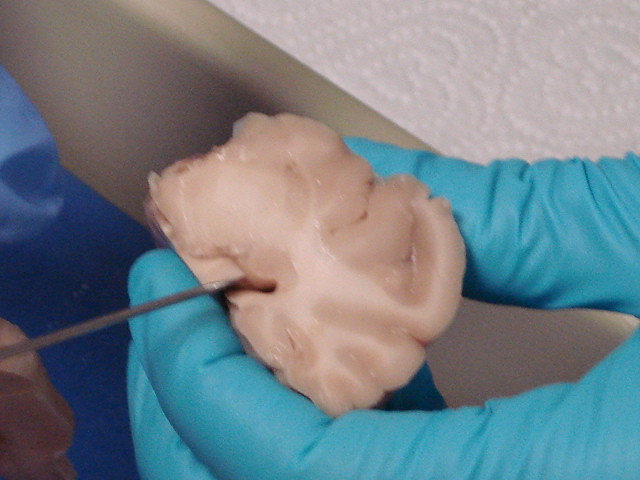The photograph captures a blurred yet intricate scene seemingly focused on a piece of dissected brain tissue held by a left hand clad in a powdered blue latex glove. The hand holding the brain prominently occupies the lower half of the frame, with only three fingers visible. The center of the image spotlights the brain tissue, distinguished by its characteristic folds and a mix of gray and white matter. A metal probe punctures the tissue from the left, trailing off beyond the frame. In the upper right corner, a paper towel with a heart design is noticeable, while a dark blue surface underneath suggests a covered table or examination area. Additional details include a faint gray border, potentially part of a box or container, running diagonally across the middle of the photograph, contributing to the overall clinical and scientific ambiance of the scene.